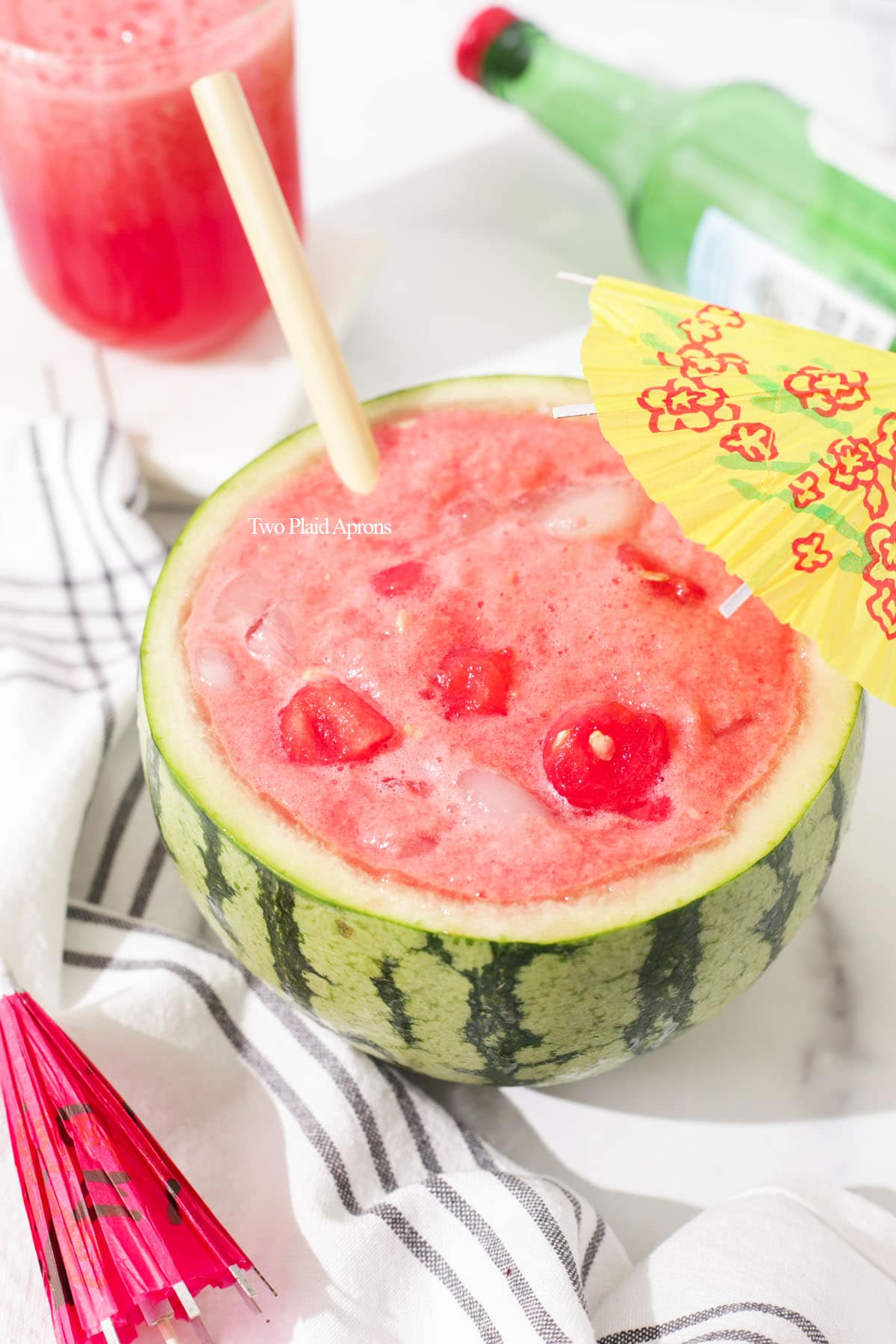This indoor photograph features a captivating and refreshing beverage served innovatively. Central to the image is a small watermelon, halved and hollowed out to serve as a unique drinking vessel. The watermelon drink inside is a vibrant, pinkish-red smoothie, teeming with foam and tiny watermelon chunks, exuding a hydrating appeal. A thick white disposable straw with yellow bands is positioned on the left, while a cheerful yellow paper umbrella adorned with red flower petals and green stripes punctuates the right.

Surrounding the watermelon drink is a mildly wrinkled white tablecloth patterned with grey horizontal and criss-crossing stripes, lending a casual touch. In the lower-left corner lies a folded pink paper cocktail umbrella with black markings, and above it, in enlarged text, "two plaid aprons" is discernible near the straw.

Further contributing to the scene, a green wine bottle with a red cap rests horizontally in the upper right-hand corner, slightly out of focus. The upper left boasts a glass pitcher, half-filled with the same red smoothie, suggesting that there’s more of the delightful concoction to enjoy. 

Overall, the photograph exudes a sense of refreshment and novelty, inviting viewers to indulge in the delightfully presented watermelon drink.